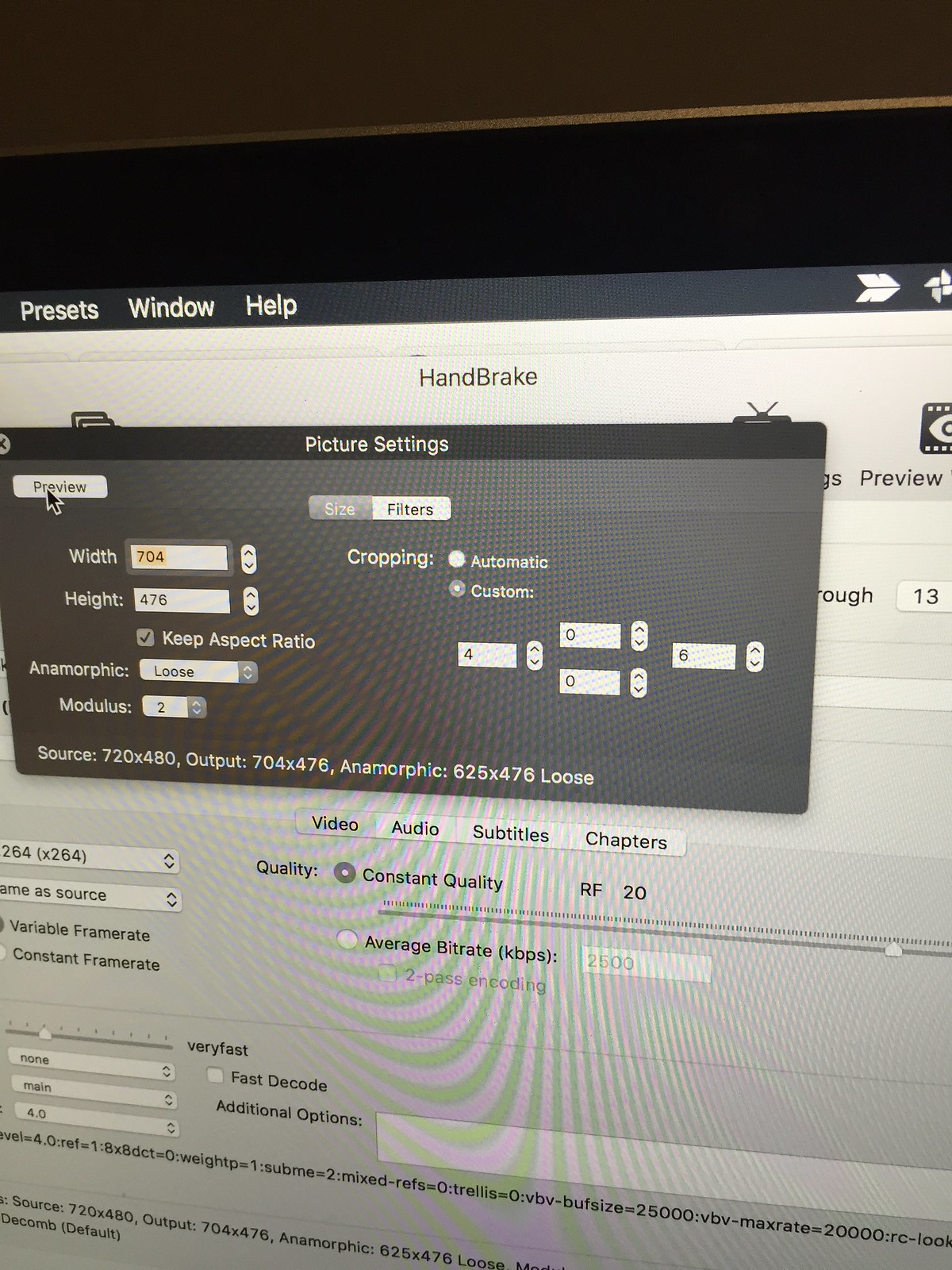The image depicts a computer screen displaying the Handbrake software interface. At the top of the screen, three menu options are visible: "Presets," "Window," and "Help." Below this, the title "Handbrake" is prominently displayed. A central black and gray pop-up titled "Picture Settings" is open, featuring a tab labeled "Preview." 

Inside the pop-up, various configuration sections are evident. The center displays options for adjusting "Size" and "Filters," while to the left, parameters such as "Width" (704 pixels), "Height" (476 pixels), "Anamorphic," and "Modules" are listed. Each parameter has adjustment buttons, and a checkbox feature for "Keep Aspect Ratio" is marked.

Below this, the pop-up contains four additional tabs: "Video," "Audio," "Subtitles," and "Chapters." A section for "Quality" settings is present, showing a checked option for "Constant Quality RF 20," and another option for "Average Bit Rate." Further down, more technical specifications can be seen, including "Source: 720x480," "Output: 704x476," and an "Anamorphic: 625x476 Loose" setting. The screen includes various settings and text fields for more detailed configurations, indicative of the user customizing video size and format settings using Handbrake.